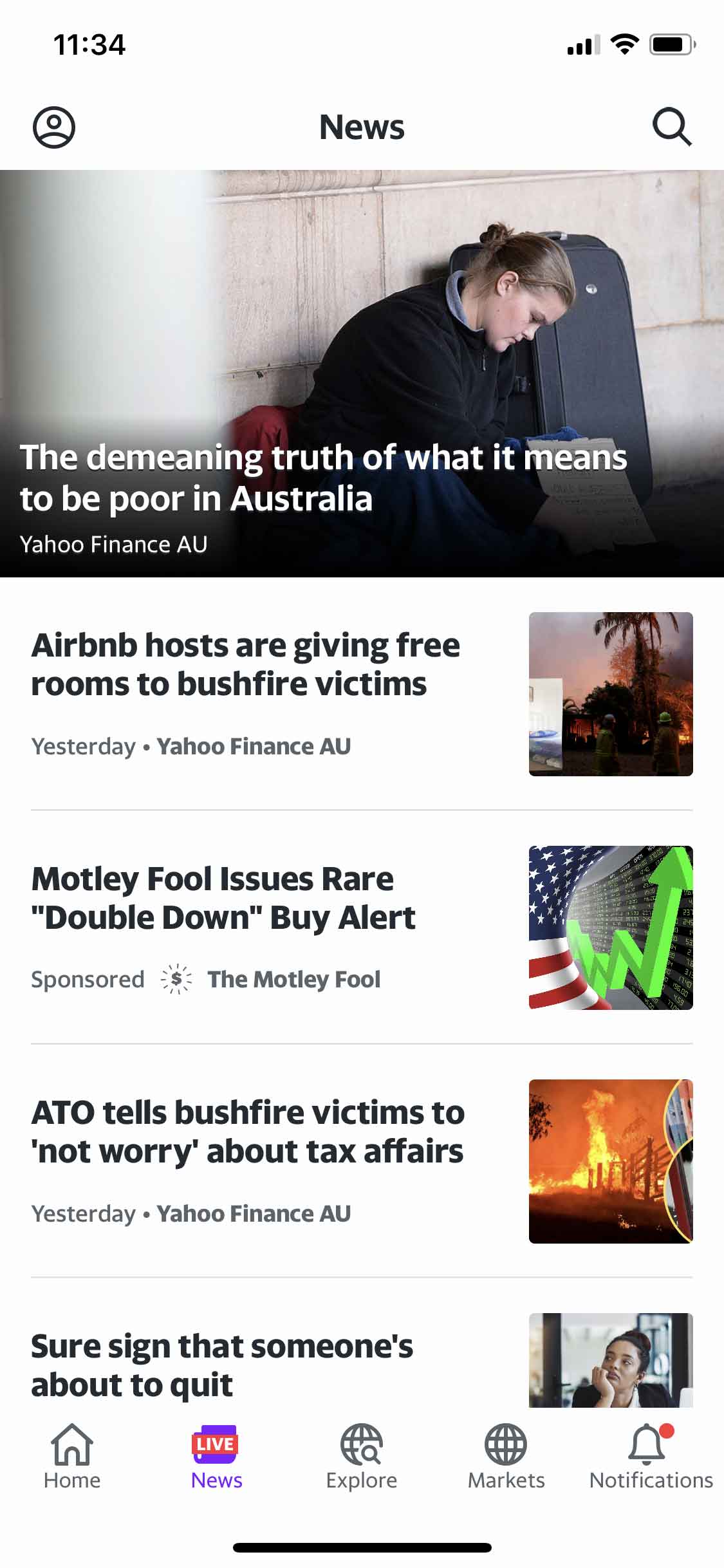Screenshot of Yahoo News Feed on a Mobile App Interface

The screenshot captures a section of a news feed from the Yahoo Australia mobile app. Dominating the top portion is a poignant photo of a woman with a downtrodden expression, accompanied by the headline, "The meaning and truth of what it means to be poor in Australia." This image sets a somber tone, highlighting the struggles faced by impoverished individuals in the country.

Below this feature article are four additional news items:

1. **Airbnb Hosts Offering Free Rooms to Bushfire Victims**:
    - This article, accompanied by a small photo of palm trees, details how Airbnb hosts are providing free accommodation to those affected by bushfires.

2. **Motley Fool Issues Rare Double Down Buy Alert**:
    - Positioned next to a generic graphic of a flag intertwined with a line graph, this article discusses a rare financial alert issued by Motley Fool, urging investors to take notice.

3. **ATO Advises Bushfire Victims to Not Worry About Tax Affairs**:
    - Featuring a photo of an intense wildfire, this article reassures bushfire victims that the Australian Taxation Office (ATO) is extending leniency regarding their tax obligations during the crisis.

4. **Sure Sign That Someone's About to Quit**:
    - Displaying an image of a woman in a contemplative pose, this piece explores the subtle indicators that an employee may be on the brink of resigning.

The screen also includes a navigation header at the top with a search box on the left and a profile icon on the right. At the bottom of the screen, icons for Home, News, Explore, Markets, and Notifications provide quick access to different sections of the app. The vertical layout and interface elements indicate its design for mobile users.